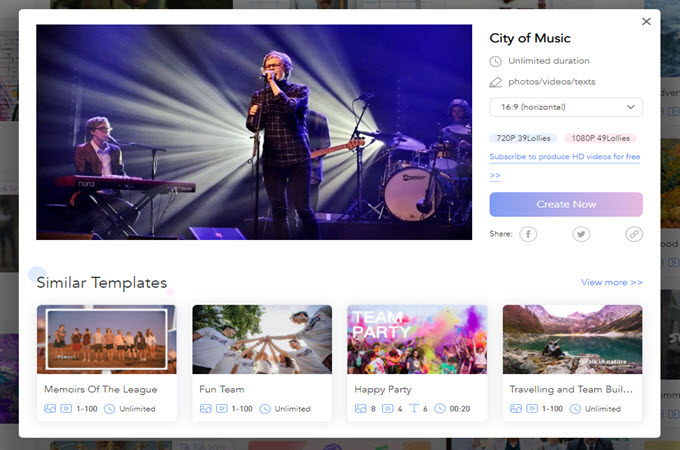**Caption:**

The image showcases a web page featuring various templates for website creation. The main focus is on a prominent overlay pop-up, partially obscuring the view of the underlying site. This pop-up has a semi-transparent gray film giving a glimpse of the content beneath. 

In the visible portion of the template, a vibrant scene depicts musicians performing: a singer (possibly a man), a pianist, and a drummer. The headline reads "City of Music" followed by "unlimited duration, photos, videos, text, 16:9 horizontal," accompanied by a drop-down menu with options such as "72 OP, 39 lollies" and "108 OP, 49 lollies."

The pop-up encourages visitors to "subscribe to produce HD videos for free" with a prominent "Create Now" button that transitions from blue to pink upon hovering. 

Below this main section are thumbnail previews of other templates labeled with titles like "Memoirs of the League," "Fun Team," "Team Party," "Happy Party," and "Traveling and Team Build" (note: "Build" appears to be misspelled as "B-U-L-I-I-L"), each indicating an "unlimited" duration and supporting content for a range of team and event-based themes.